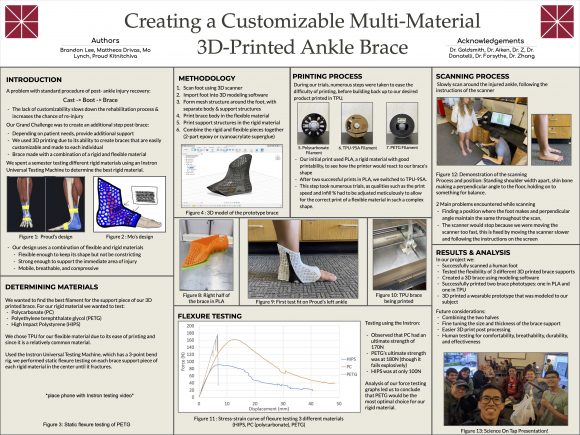This detailed diagram, seemingly from a book or a PowerPoint presentation, measures approximately five inches wide by three inches high. It features a white header spanning the top, adorned with red triangles in each corner forming squares with white starburst patterns inside. Dominating the header in bold black font is the title, "Creating a Customizable Multi-Material 3D Printed Ankle Brace." The left section of the header lists the authors, although they are partially blurred and difficult to read, with "Bradley Matthews" discernible. The right section contains acknowledgements.

Beneath the header, the background transitions to a light tan color, segmented into multiple rectangles that provide a comprehensive breakdown of the project. The first rectangle, positioned at the top left, is labeled "Introduction" and includes images of a human calf and foot fitted with a blue ankle brace. Below this, the section titled "Determining Materials" delves into the components used for the brace. The "Methodology" section, to the right, features a computer graph detailing the development of the brace, followed by the "Printing Process" on the right side, explaining the actual 3D printing steps involved.

The "Flexure Testing" section below "Methodology" contains a graph measuring the ankle brace's flexibility. To the right, the "Scanning Process" box displays an image of a man and woman examining a brace on an ankle. In the bottom right-hand corner, the "Results and Analysis" section is highlighted by a team photo of the smiling project members, indicating collaborative effort.

Included in the visuals are varied objects like people, computers, an ankle brace, and a 3D printer, with colors spanning red, white, green, black, blue, orange, and purple. Despite some text being too small to read, the legible portions caption a step-by-step guide to creating the 3D printed ankle brace, detailing every phase from introduction and material selection to final results and team acknowledgment.